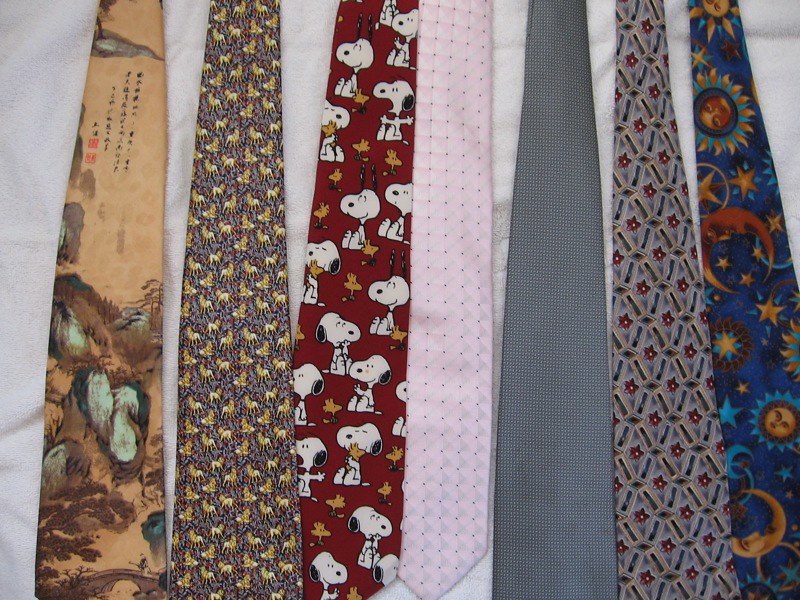This is a photograph of seven ties, each distinct in design and neatly arranged side-by-side on a white blanket. The ties are displayed vertically from left to right. The first tie features light brown with Japanese art depicting vertical black kanji characters beside illustrations of trees and leaves. Next, a tie with a pattern of small, intricately arranged lines in mixed patterns of gold, blue, and red. The third tie stands out with vibrant red featuring repeating images of Snoopy and Woodstock from the Peanuts comic strip. The fourth tie is simple, white adorned with black dots. Moving along, the fifth tie is dark blue, dotted with very tiny white spots. The sixth tie showcases a formal, floral and geometric pattern with red flowers set against a dark blue, gold-accented background. Finally, the seventh tie on the far right is adorned with a celestial theme, including suns, moons, and stars in dominant tones of dark blue, gold, and orange, with detailed faces on the sun and crescent moon.